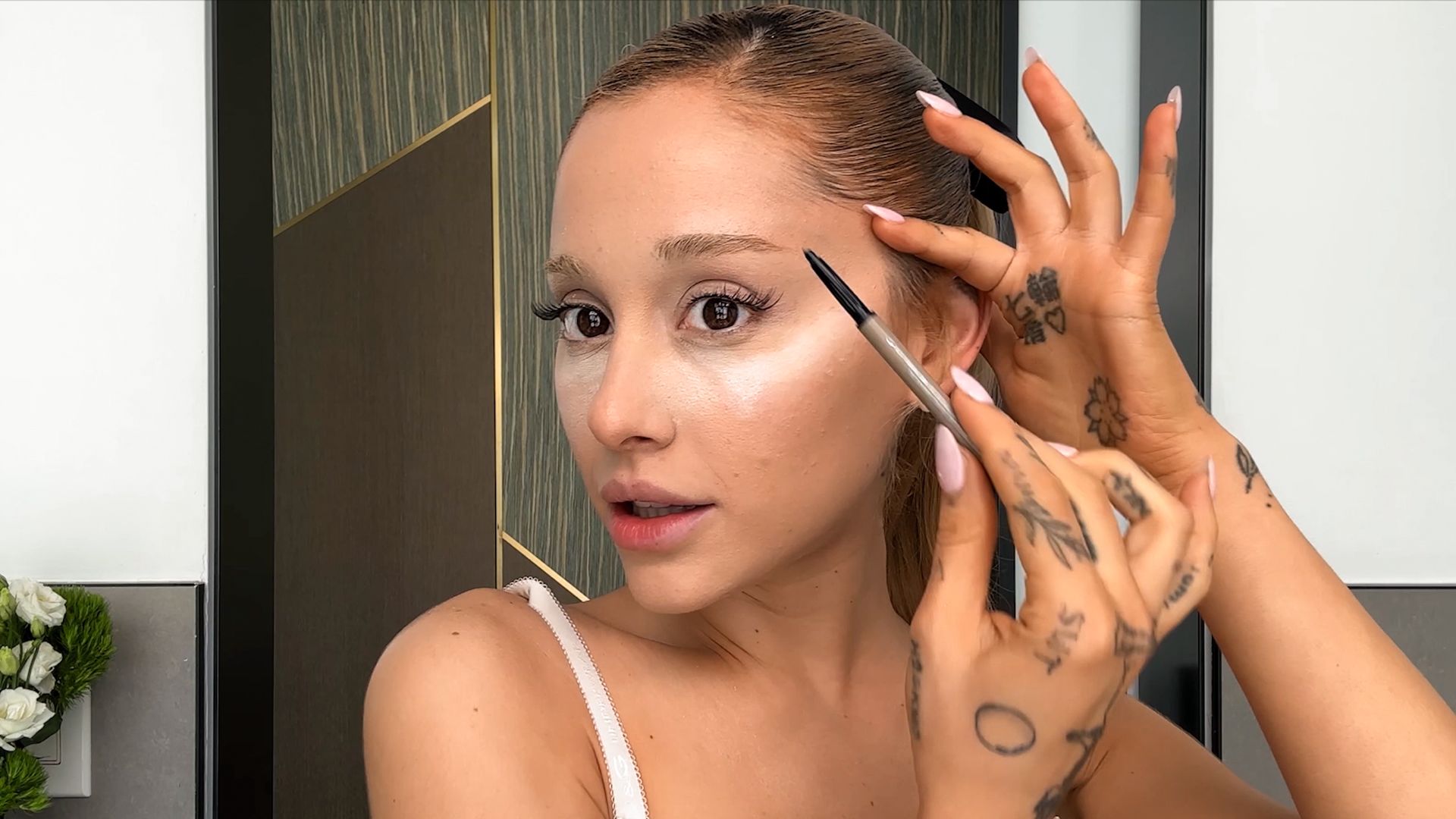The photo showcases a young woman, likely in her 20s or 30s, applying makeup in front of a mirror. She has brown hair pulled back into a ponytail and tanned skin with a smooth complexion. She is in the process of applying eyeliner and has already worked on her eyelashes and brows, giving careful attention to detail. Her thin eyebrows are neatly shaped, and her eyelashes appear to be curled upwards. She has some white reflective makeup under her eyes, enhancing her cheekbones. Her hands, which are adorned with multiple tattoos, including flowers, circles, Chinese characters, and other designs, also display pink nail polish. She wears a tank top, and although the exact setting is unclear, the background features a white wall with green wooden paneling, suggesting a well-decorated space. The woman is looking directly into the camera while concentrating on her makeup application, presenting herself with precision and care. The blend of her artistic tattoos and polished look suggests a unique and confident personal style.